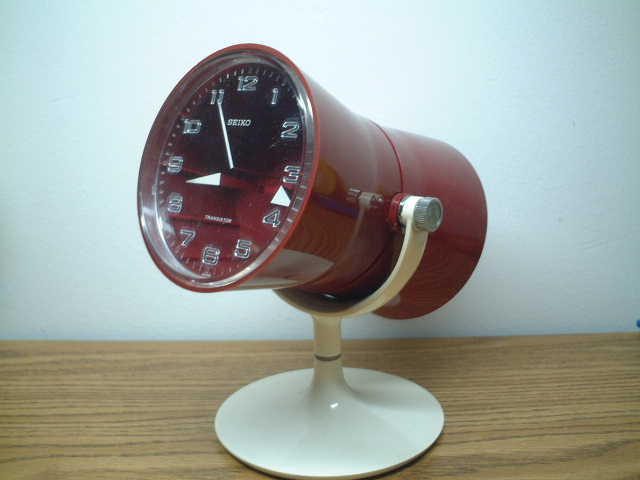This photograph features a red clock mounted onto a decorative object typically used for hanging mirrors. The base of this decorative object is white, contrasting sharply with the crimson clock. The clock face indicates the time as approximately 8:55. It is positioned on a circular wooden table, adding a rustic charm to the scene. The background is a plain white wall, creating a neutral backdrop that accentuates the vivid colors of the clock. The clock is secured to its base with two prominent screws. In the middle right-hand corner of the image, a small portion of another unidentified object is visible, hinting at more elements outside the frame. The orientation of the clock suggests it is slightly skewed to the left, pointing in a northwest direction.